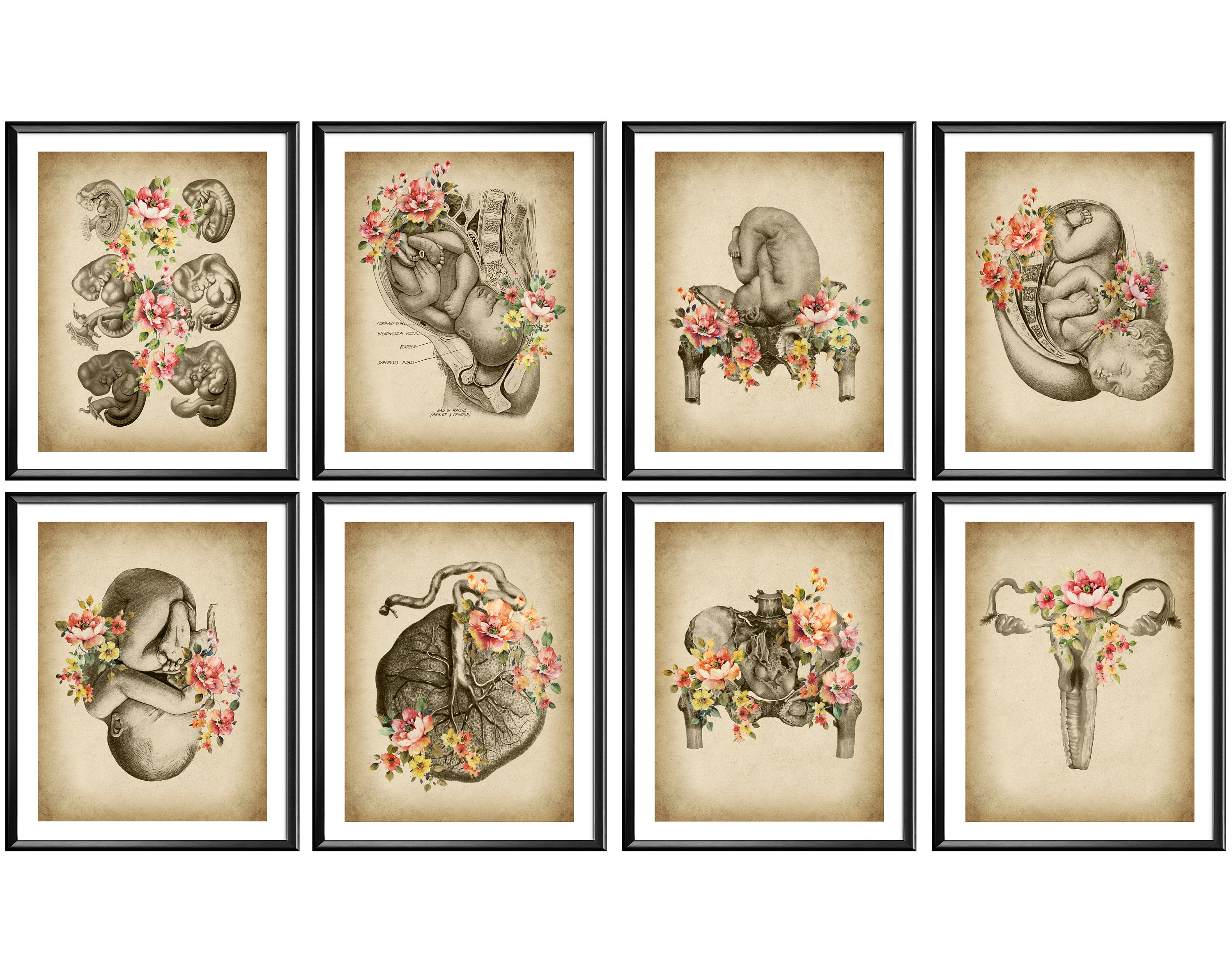This image captures a set of intricate artworks themed around pregnancy and childbirth, displayed in a grid with four columns and two rows. Each artwork is framed in a thin black frame with white matting, set against a tan or brownish background that gives the paper a vintage, slightly dirty appearance. The drawings, executed in black and brown lines, depict various stages and elements of pregnancy, including fetuses at different stages, the uterus, the placenta, and scenes of childbirth. While the detailed line work focuses on anatomical accuracy, each piece is embellished with vibrant floral designs in pinks, yellows, and oranges, adding a striking contrast to the monochromatic drawings. The floral accents seem to drape and intertwine with the anatomical elements, highlighting the fusion of natural beauty and biological processes. Despite the small size of the images, which makes it difficult to discern all details, the colorful flowers are particularly eye-catching against the subdued backgrounds.